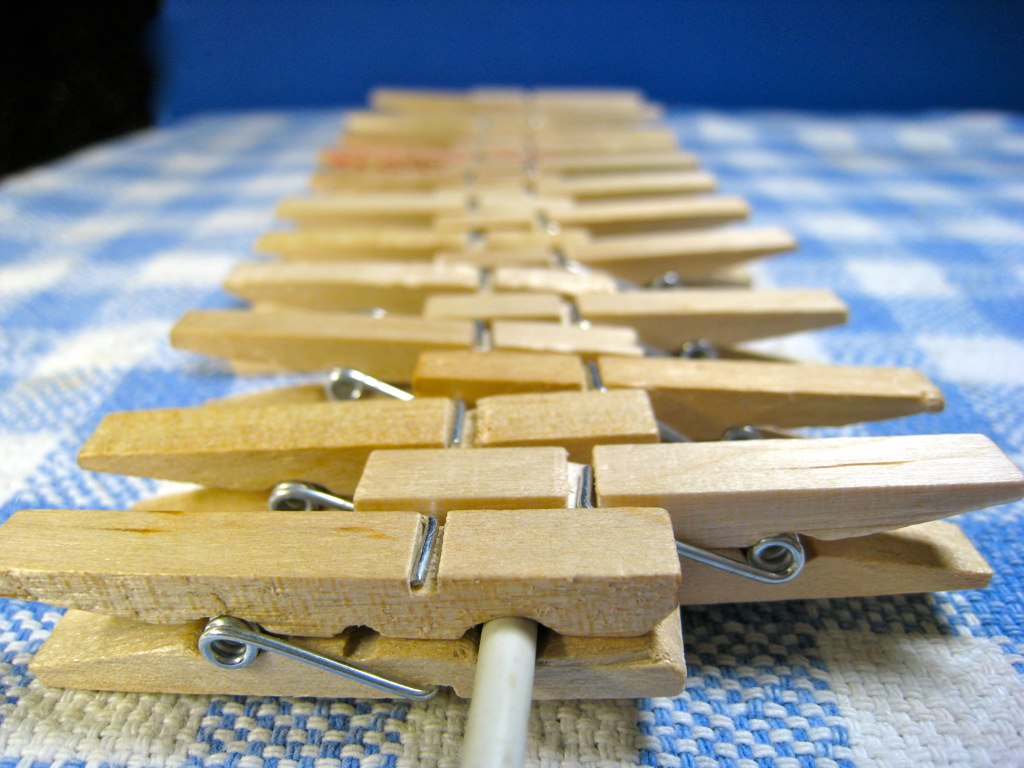The image is a highly detailed, close-up shot featuring a long line of wooden clothespins clamped onto a white wire. The clothespins are positioned in an alternating pattern, with the first one facing left, the next facing right, and continuing this pattern throughout, giving them the appearance of a zipper extending into the background. The scene is set on top of a blue and white checkered blanket, almost resembling a picnic cloth. The photograph captures the clothespins from a low-angle perspective, showcasing their metallic spring mechanisms clearly. The shallow depth of field brings the foremost clothespins into sharp focus, while those in the background gradually blur. Off in the distance, the dark blue wall provides a contrasting backdrop that accentuates the clothespins' wooden texture and the white wire they cling to. There are approximately 30 to 40 clothespins in the shot, each aligned meticulously, stretching horizontally across the image.